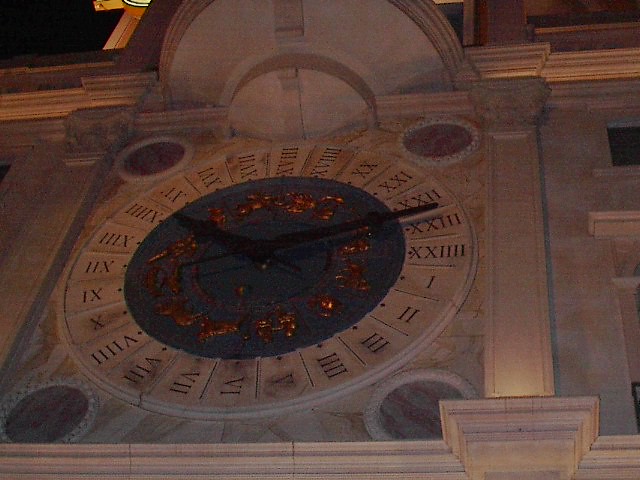This image features a unique clock that diverges from conventional designs. Unlike a typical 12-hour clock, this timepiece displays a full 24 hours on its face. Additionally, the arrangement of the numbers is unconventional; instead of starting at the top, the sequence begins on the right side of the clock. This atypical setup gives the clock a distinctive and intriguing appearance, setting it apart from ordinary timekeeping devices.